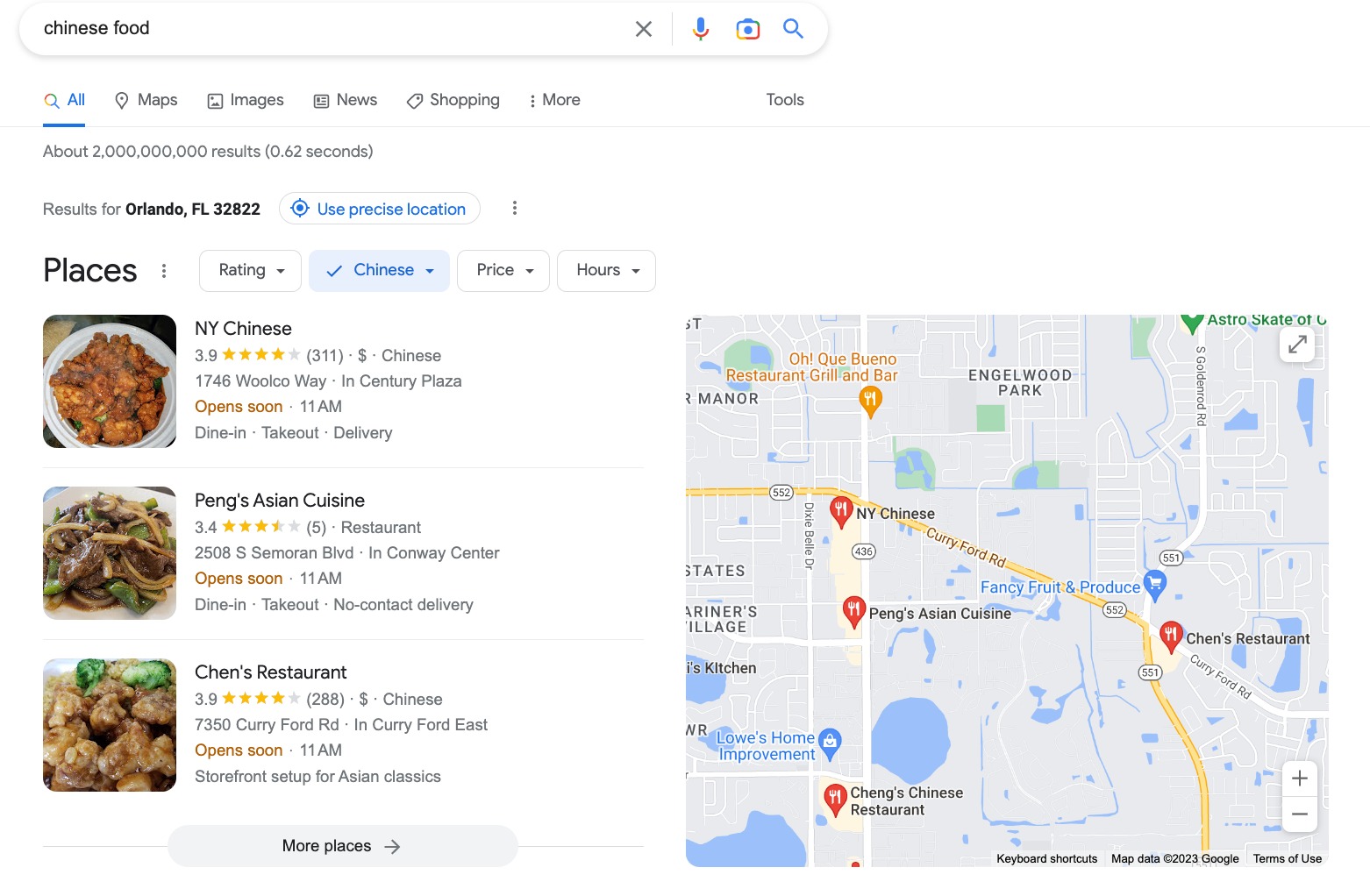The photograph depicts a detailed search query interface on a white background, presented in portrait orientation. At the top, there is an oval-shaped white search bar with "Chinese food" typed in black font on the left side. Below the search bar, the interface provides filtering options including "All," "Maps," "Images," "News," "Shopping," and "More," with the "All" category currently selected. To the right, there are additional filter tools. The search results indicate that approximately 2 billion results were found in 0.62 seconds, tailored specifically for the location "Orlando, Florida 32822," with an option to use precise location for more accurate results.

Beneath this, the section labeled "Places" offers further filters such as rating, type (with "Chinese" already selected and checked), price range, and hours of operation. This section also includes images and brief descriptions for three prominent options:

1. **NY Chinese** - Featuring an image of a plate with a brown food item.
2. **Peng's Asian Cuisine** - Displaying a dish that appears to contain meat, noodles, and vegetables.
3. **Chen's Restaurant** - Showcasing what looks like glazed chicken.

On the right side of this section, there is a square map illustrating the locations of these restaurants, showing their proximity to each other with labeled pins for easy identification.